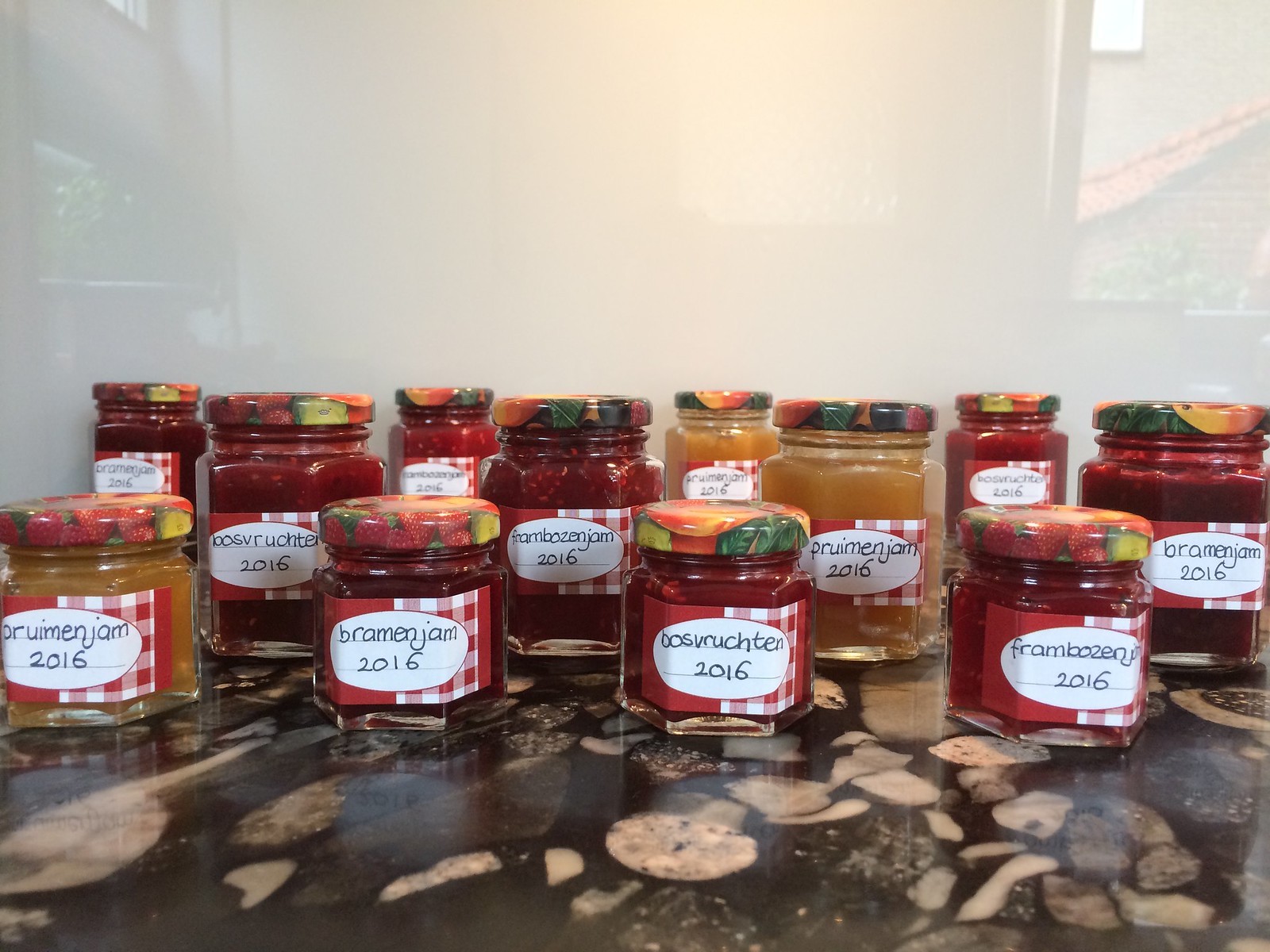The image is an indoor color photograph featuring a meticulously organized collection of jam jars placed on a dark marble countertop, against a white background. These jars, twelve in total, are arranged in three neat rows of four, with the front row's jars appearing shorter than those in the middle and back rows, allowing full visibility of all labels. The jars are octagonal in shape and made of glass, each topped with a colorful screw-type lid adorned with illustrations of fruits like strawberries and peaches. The red and white labels on the jars are consistent, featuring a red left side and a red and white gingham pattern on the right, with a white oval in the center containing handwritten descriptions of the jam and the date, which is uniformly 2016. The labels feature names such as "Bramble Jam," "Bosh Rush Jam," "Farm Boys Jam," and "Fram Bros Jam." The jams inside vary in color, suggesting different flavors, and each jar appears completely filled to the top. The dark marble countertop, detailed with light brown spots, enhances the aesthetically pleasing presentation of the colorful jam assortment.